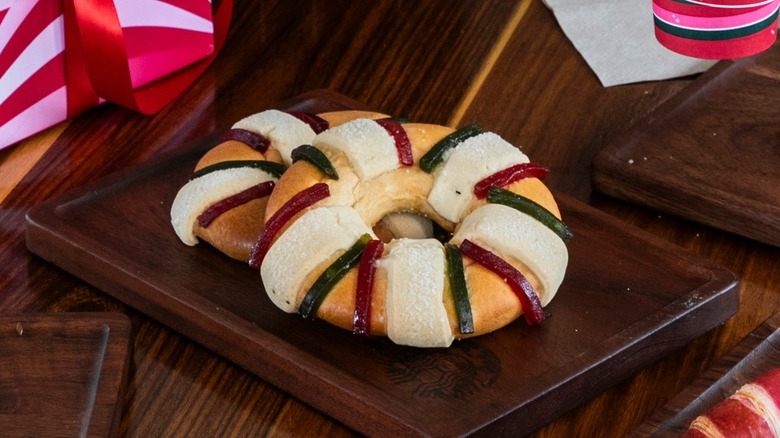This photograph showcases a pair of sweet treats, identified as Three Kings bread, displayed elegantly on a dark brown wooden serving board which features a faint Starbucks logo in the bottom right corner. These dessert items, similar in size to bagels, have a medium to light tan hue. Each piece is adorned with five prominent white frosting stripes that start in the center and cascade over the edges, complemented by smaller stripes of dark green and red icing, which appear slightly translucent and jelly-like. The breads are stacked, with one resting slightly atop the other. The serving board is placed on a dark brown, wood-grain table, adding a rustic charm to the presentation. In the background, the scene includes a partially visible red and white package with a pink stripe and a red ribbon, along with a glimpse of a red Starbucks cup sitting on top of a napkin in the top right corner.